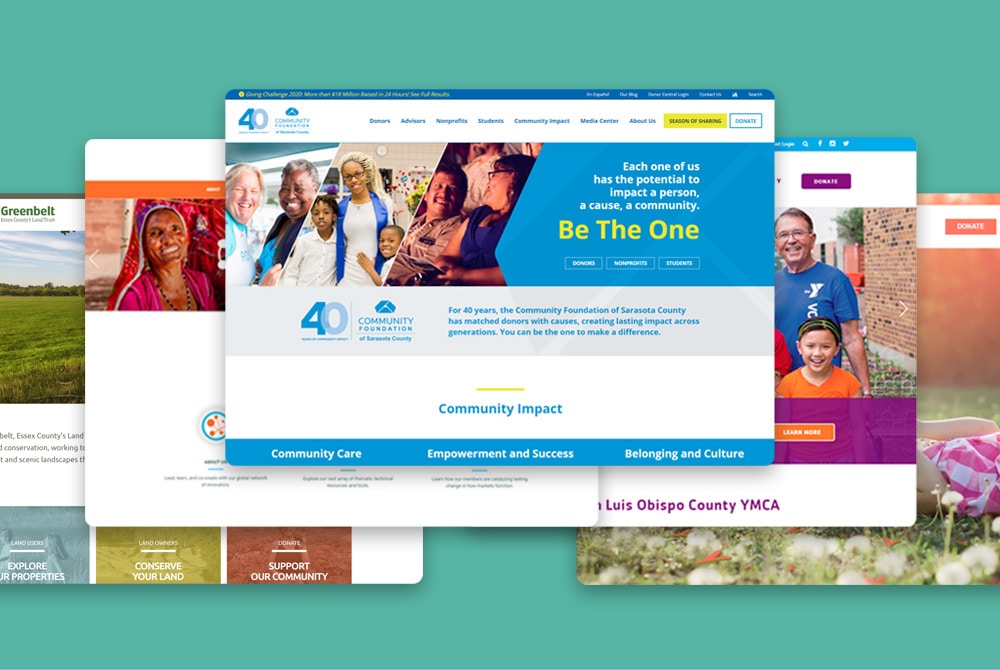The image displays a website with a landscape orientation, featuring a matte turquoise or teal green background. Superimposed on the background are multiple web screen thumbnails. 

At the top of the image, there is a prominent web screen displaying three photographs of diverse individuals laughing and smiling. Accompanied by the text, "Each one of us has the potential to impact a person, a cause, a community. Be the one," this section promotes a powerful message of community involvement. Below this text, there are several buttons, although their labels are unreadable.

Further down, a segment reads "40 Years of Community Impact," highlighting the organization's longstanding commitment. At the bottom of the screen, clickable options read: "Community Care," "Empowerment and Success," and "Belonging and Culture," serving as navigation links to different sections of the website.

To the right, there's another web screen featuring the San Luis Obispo County YMCA. It includes a photograph of a dad wearing a blue YMCA shirt, standing next to his child in front of a brick building.

On the left side, an older woman dressed in traditional attire suggests a potential focus on international outreach or multicultural engagement, possibly still under the YMCA umbrella.

The final web screen, labeled "Greenbelt," showcases an agrarian field, hinting at an agricultural or environmental nonprofit.

Overall, the image represents various nonprofit organizations, emphasizing themes of community, diversity, and collective impact.